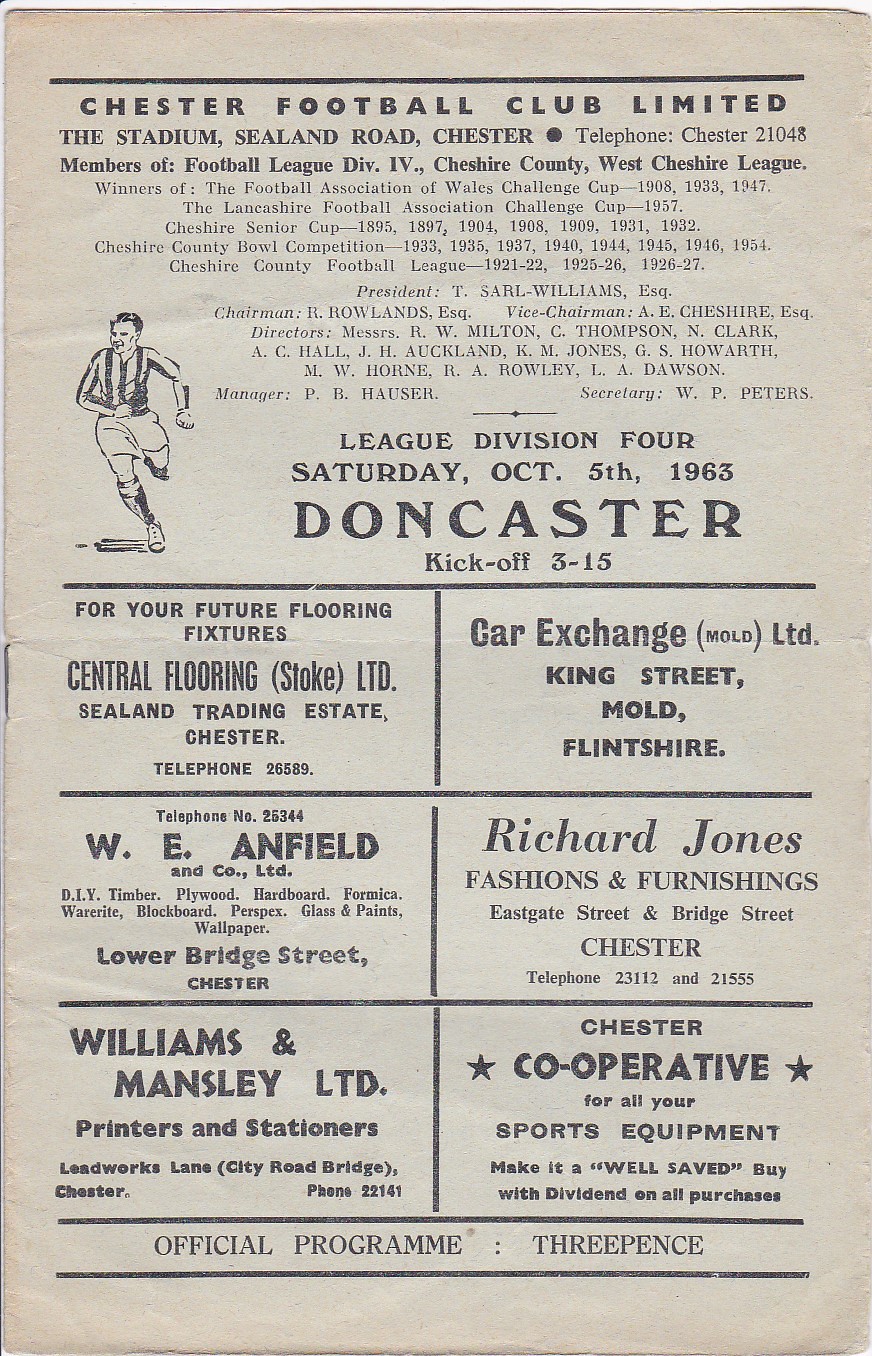The image is of a weather-worn, vintage program or advertisement for Chester Football Club Limited. At the top, a horizontal black line borders bold black text reading "Chester Football Club Limited, The Stadium, Sealand Road, Chester, Telephone Chester 21048." The next lines detail the club's membership in the Football League Division IV, Cheshire County, and West Cheshire League, along with numerous accolades, such as winners of the Football Association of Wales Challenge Cup in 1908, 1933, and 1947, among other titles. Leadership is also listed, including President T. Sarle-Williams, Esquire, and Chairman R. Rowland, Esquire. 

To the left of this text, there's an illustration of a man in a black and white uniform, assumed to be a soccer player, running. The player wears a long-sleeve striped shirt, shorts, knee-high socks, and tennis shoes. Below, in bold print, the event details read: "League Division IV, Saturday, October 5th, 1963, Doncaster, Kickoff 3-15."

The bottom section consists of six advertisement squares. The top-left ad is for Central Flooring, Stoke LTD, Sealand Trading Estate, Chester, Telephone 26589. Adjacent to this, Car Exchange, LTD, King Street, Mold, Flintshire, is listed. The middle-left ad provides the contact for W.E. Anfield and Company, LTD, Lower Bridge Street, Chester, advertising DIY materials and featuring a telephone number 25344. Next to it, an ad for Richard Jones, Fashions and Furnishings, Eastgate Street and Bridge Street, Chester, with telephone numbers 23112 and 21555. The lower-left ad belongs to Williams and Mansley, LTD, Printers and Stationers, Leadworks Lane, City Road Bridge, Chester, Telephone 22141. The final, right-hand ad promotes Chester Cooperative for all sports equipment with the slogan "Make It a Well-Saved Buy With Dividend on All Purchases." 

At the base, the program concludes with the statement "Official Program, 3 pence" bordered by another horizontal line.